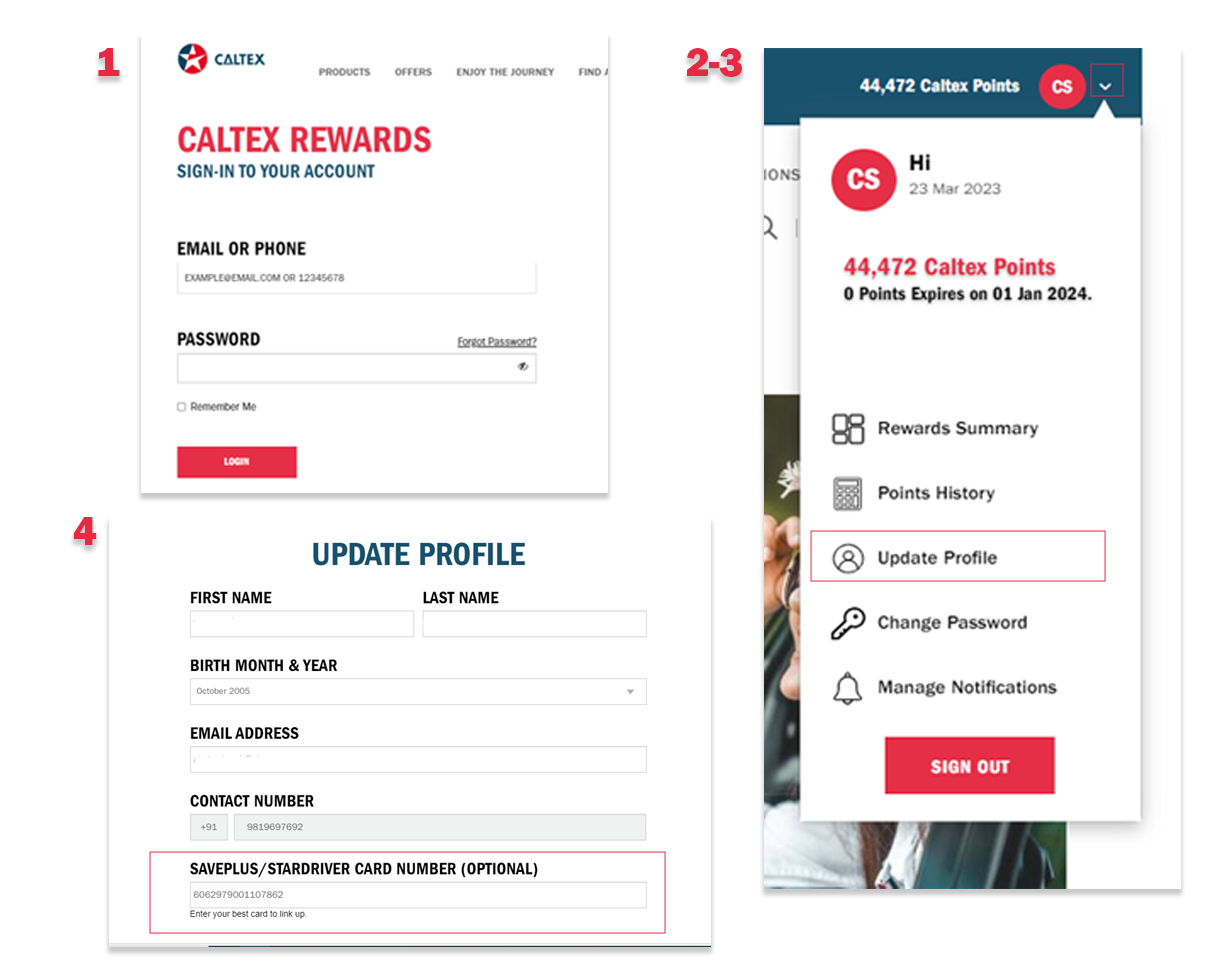This detailed image showcases a web page interface with three distinct windows, primarily associated with Caltex:

1. **Login Window (Left side)**
   - **Company Name and Logo**: The top left corner features the "Caltex" name and logo.
   - **Menu Bar**: Adjacent to the logo, the menu starts with options like "Products," "Offers," and "Enjoy the Journey."
   - **Special Highlight**: The page prominently displays "Caltex Rewards" in red text with a green "Sign into your account" prompt beside it.
   - **Login Fields**: 
     - **Email/Phone Field**: A place to enter your email or phone number.
     - **Password Field**: Includes a toggle-able eye icon for password visibility.
   - **Extra Links and Options**:
     - "Forgot password" link above the password field.
     - "Remember me" checkbox under the password field.
     - **Login Button**: Positioned at the bottom left corner, in red.

2. **Profile Window (Center)**
   - **Avatar and Introduction**: A red circle avatar with "CS" initials introduces the user "Hi, posted 23," a member since March 23, 2023.
   - **Caltex Points**: Displaying a total of 44,472 points.
   - **Profile Menu**:
     - **Reward Summary**: Icon listed.
     - **Points History**: Icon listed.
     - **Update Profile**: Icon represented by a silhouette avatar.
     - **Change Password**: Indicated with a key icon.
     - **Manage Notifications**: Showcased with a bell icon.
   - **Sign Out Button**: Situated in red at the bottom of the profile section.

3. **Update Profile Window (Bottom left, white)**
   - **Title**: "Update Profile" centered at the top.
   - **Profile Sections**:
     - First Name
     - Last Name
     - Birth Month and Year
     - Email Address
     - Contact Number
     - **Safe Plus/Star Driver Card Number (optional)**: This section is marked in red.

This detailed caption elucidates the organization and specific features within each window, highlighting the various interactive elements and design aspects of the Caltex web page.